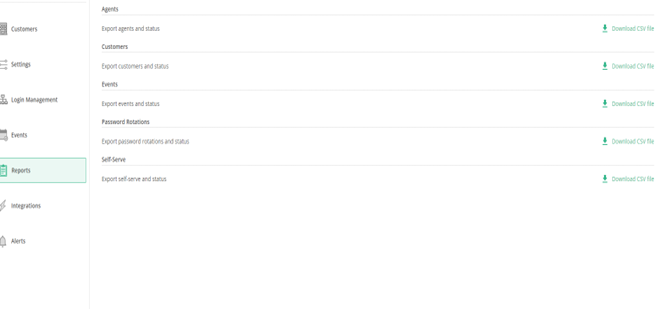The image is a small, drab, and primarily monochromatic screenshot of a web page set against a white background. The text is rendered in light gray, making it difficult to read. On the left side, there is a vertical navigation menu with sections labeled "Customers," "Settings," "[Unclear] Management," "Events," "Reports." Each of these sections is highlighted with a green background and green trim, which adds a slight contrast to the otherwise muted palette. 

To the right, the main content area is headed with "Agents," followed by several listed items such as "Customers," "Events," "Password Registration," and "Self-Service," all in very small print. Adjacent to each item on the right, there are icons indicating the option to download, visible as a green arrow. Just beneath each arrow, a green line provides additional visual separation. Text accompanying the download options reads "Download a CRV file or CTV file."

Overall, the image depicts a bland, hard-to-read web page interface with a green-accented navigation menu and download options for specific sections.